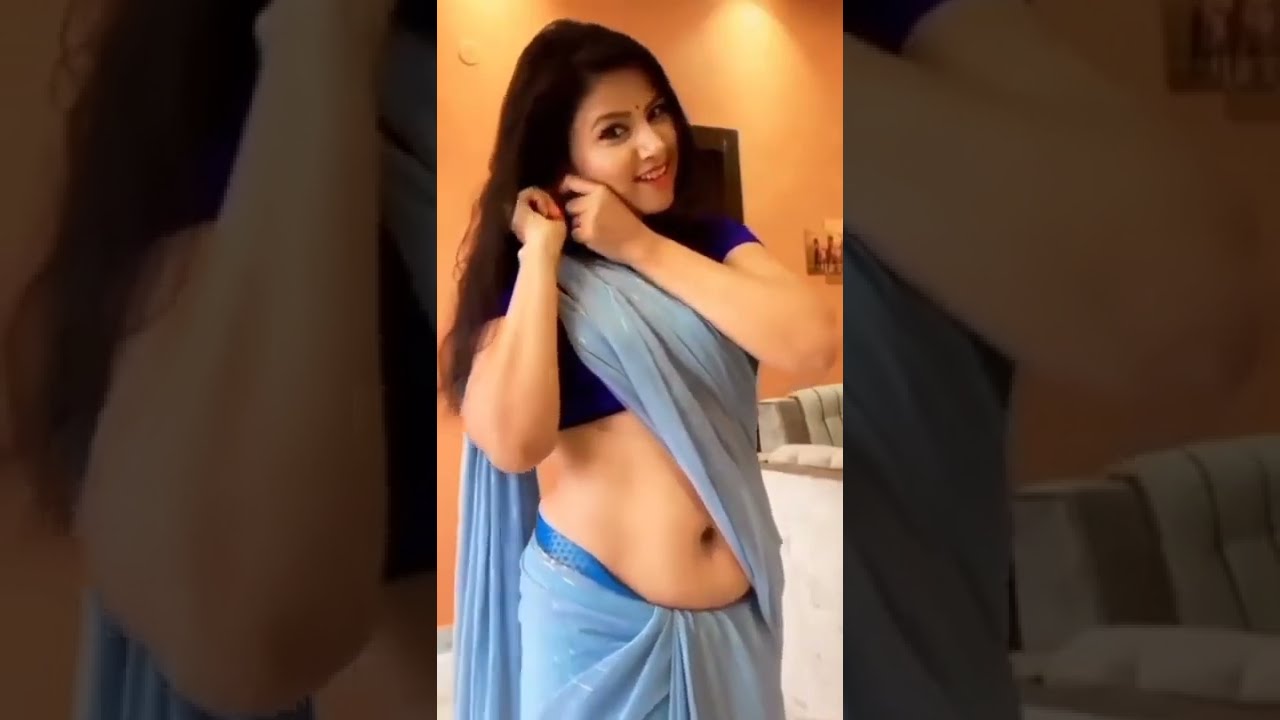The image is a detailed composite of three rectangular slides. The central slide is a clear photograph of an Indian woman standing in what appears to be a living room with a white sofa and an orange-colored wall. She has long, dark hair and a red bindi on her forehead, suggesting her cultural background. She is dressed in a traditional Hindu sari, which is light blue with a sash draped over her right shoulder, and features an exposed section on the right side of her torso. Her elbows are bent, and her hands are near her ears as if she is adjusting an earring. The slides on either side of the main image are zoomed-in, faded, and filtered versions of the same picture, with one prominently showing her bent elbow and the other being indistinct and heavily filtered. The composition lacks any text but provides a vivid depiction of the woman in her interior setting, highlighted by the vibrant colors of her attire and the warm tones of the room.